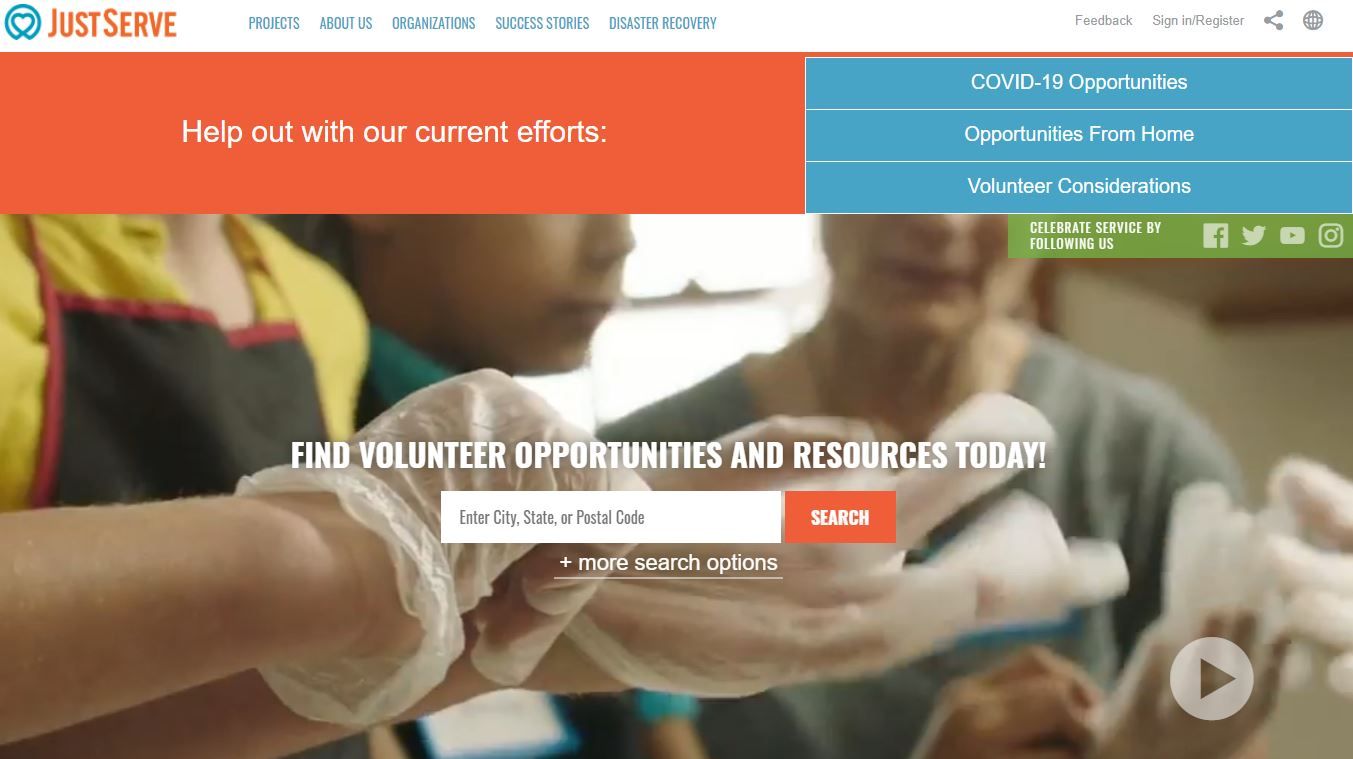This image, taken from the JustServe website, showcases the comprehensive layout and features of the platform. At the top, the navigation bar prominently displays options such as "Projects," "About Us," "Organizations," "Success Stories," and "Disaster Recovery." Additionally, users have access to "Feedback," "Sign In," and "Register" links.

Moving down the homepage, an orange box stands out with the message "Help out with our current efforts," pointing visitors towards specific initiatives like "COVID-19 Opportunities," "Opportunities from Home," and "Volunteer Considerations," each enclosed in teal boxes on the left-hand side. Directly underneath "Volunteer Considerations," there is an invitation to "Celebrate service by following us," accompanied by social media icons for Facebook, Twitter, YouTube, and Instagram.

Dominating the central section of the image, photographs depict volunteers engaged in arts and crafts activities, donning gloves and one wearing an apron, underscoring the hands-on nature of the service projects. The call to action "Find volunteer opportunities and resources today" encourages users to enter their city, state, or postal code into a search field and click the red "Search" button at the end, streamlining the process of finding local volunteering options.